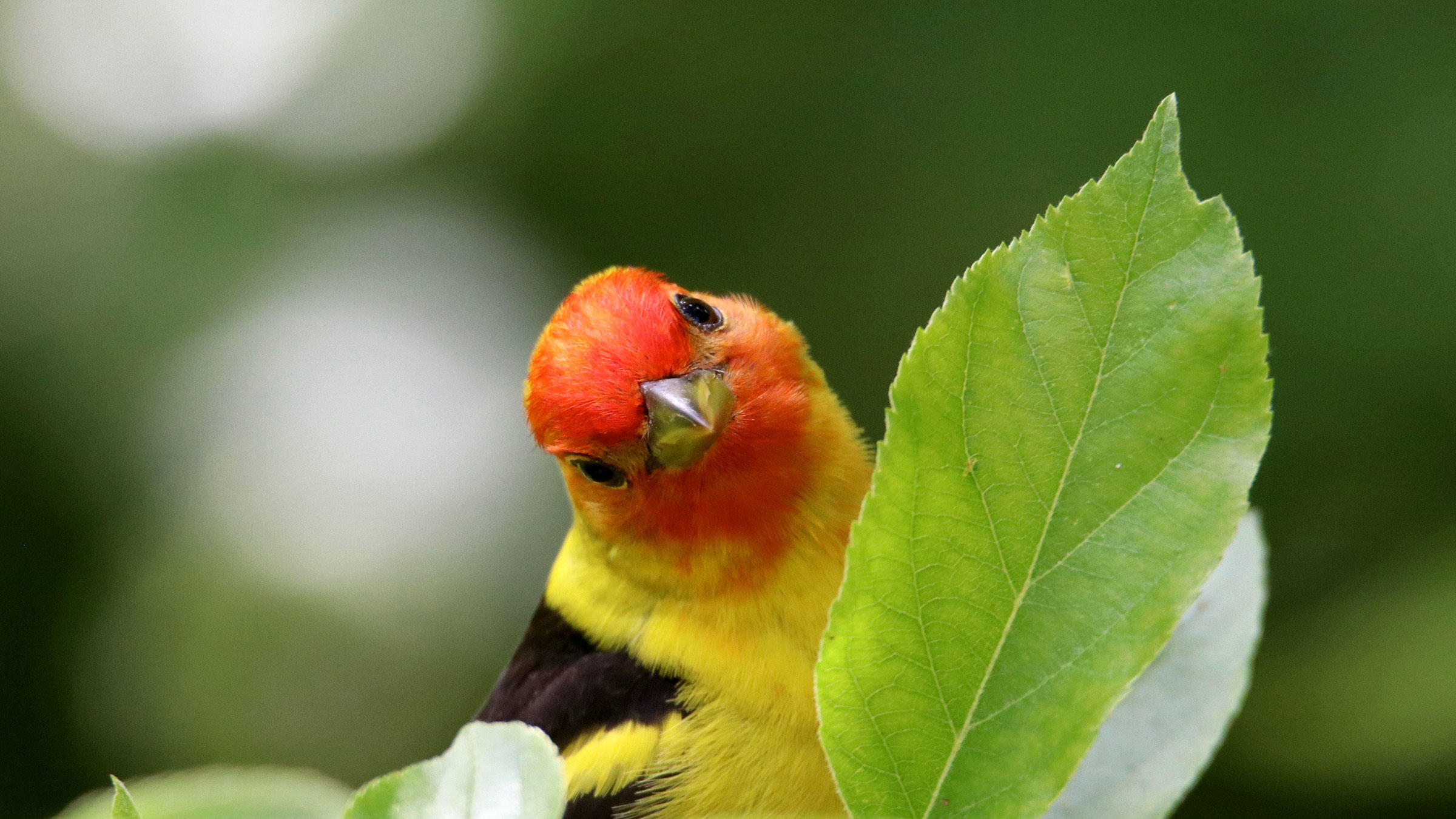The image captures a vibrant outdoor scene with a blurred hunter-green background, accentuated by bright white circles that suggest light filtering through foliage. Dominating the foreground on the right side, a singular, sharply defined green leaf with rough, zigzag edges emerges from the bottom of the frame. Partially obscured by this leaf is an eye-catching bird, which seems to face the camera with a slightly tilted head. The bird's beak is strikingly gold and pointed, measuring about an inch long. Its vivid red head extends from the beak across the top to the chest, blending into a bright yellow body. The short feathers transition to black wings with yellow tips. The bird’s large black eyes stand out, giving it an expressive look. Additional, less discernible leaves and green elements appear along the bottom and behind the bird, enhancing the natural and lively composition of the photo.